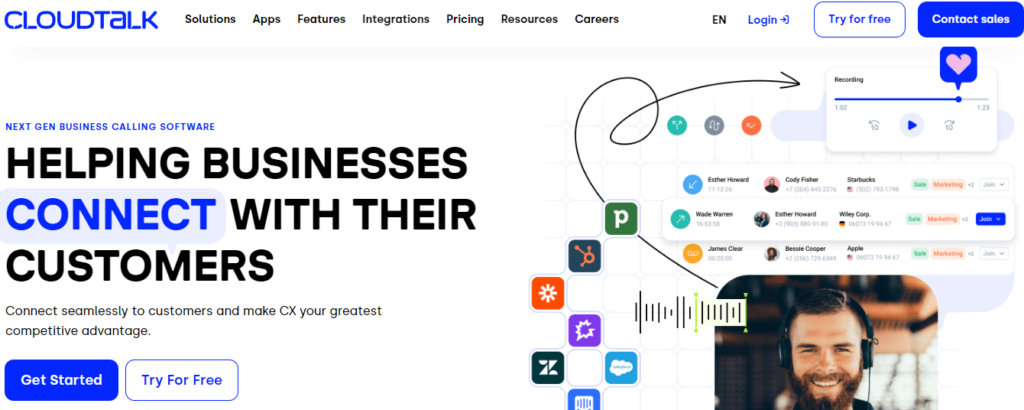The image is a screenshot of a professional website with a white background. At the top left side, the site's logo "CloudTalk" is prominently displayed in blue text. Adjacent to the logo are the navigation links written in smaller black text: "Solutions," "Apps," "Features," "Integrations," "Pricing," "Resources," and "Careers." On the top right, there is a language option indicated by "EN" in black text followed by a blue "Login" link, accompanied by an arrow pointing to a square bracket.

To the far right of the header, there are two call-to-action buttons: the first button is white with blue text, labeled "Try for Free," and the second button is navy blue with white text, labeled "Contact Sales." Beneath this header, a tagline appears in smaller capitalized letters: "NEXT GEN BUSINESS CALLING SOFTWARE." Directly below, in larger font, is the phrase "Helping Businesses Connect with Their Customers." Under this headline, there's a smaller text snippet: "Connect Seamlessly to Customers and Make CVX Your Players' Competitive Advantage."

Two more call-to-action buttons are beneath this text: a blue button with white text labeled "Get Started" and another white button with blue text labeled "Try for Free."

On the right side of the website, several images are displayed. The largest image features a fair-complexioned man with a beard wearing a headset. To the left of him, several square logos and symbols are visible. Above the man is a waveform illustration, indicative of a recording. Further above, there are small profile pictures and customer names. At the top, there is a white box labeled "Recording" with a progress bar. This progress bar includes a blue heart, a colored box, a play button, a minus 10 seconds button, and a fast-forward 10 seconds button.